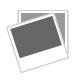The colored photograph showcases a vibrant Lego Creator product box, prominently featuring an underwater robot as the centerpiece of this kit. The packaging indicates that the set is suitable for ages 7 and up and is identified by the model number 31090. The box highlights that the kit contains 207 pieces and offers the versatility to construct three different robotic models, noted by the "3 in 1" label on the side. A small orange banner at the bottom serves as a cautionary note about the choking hazard.

The underwater robot displayed on the box is predominantly yellow with dark gray or black accents and is equipped with claw-like arms. The box also includes secondary models: a blue and white manta ray and a small green underwater plant, appearing to emerge from a minimal beige base. The background imagery is a gradient of ocean blue, transitioning to a sea-green tint towards the bottom, providing a realistic underwater setting.

Additionally, three smaller images positioned along the top of the box illustrate the alternate robotic creations possible with the included pieces. The iconic red Lego logo is clearly visible on multiple corners of the box, ensuring brand recognition. The overall background of the photograph itself is white, making the vibrant elements of the Lego box stand out.